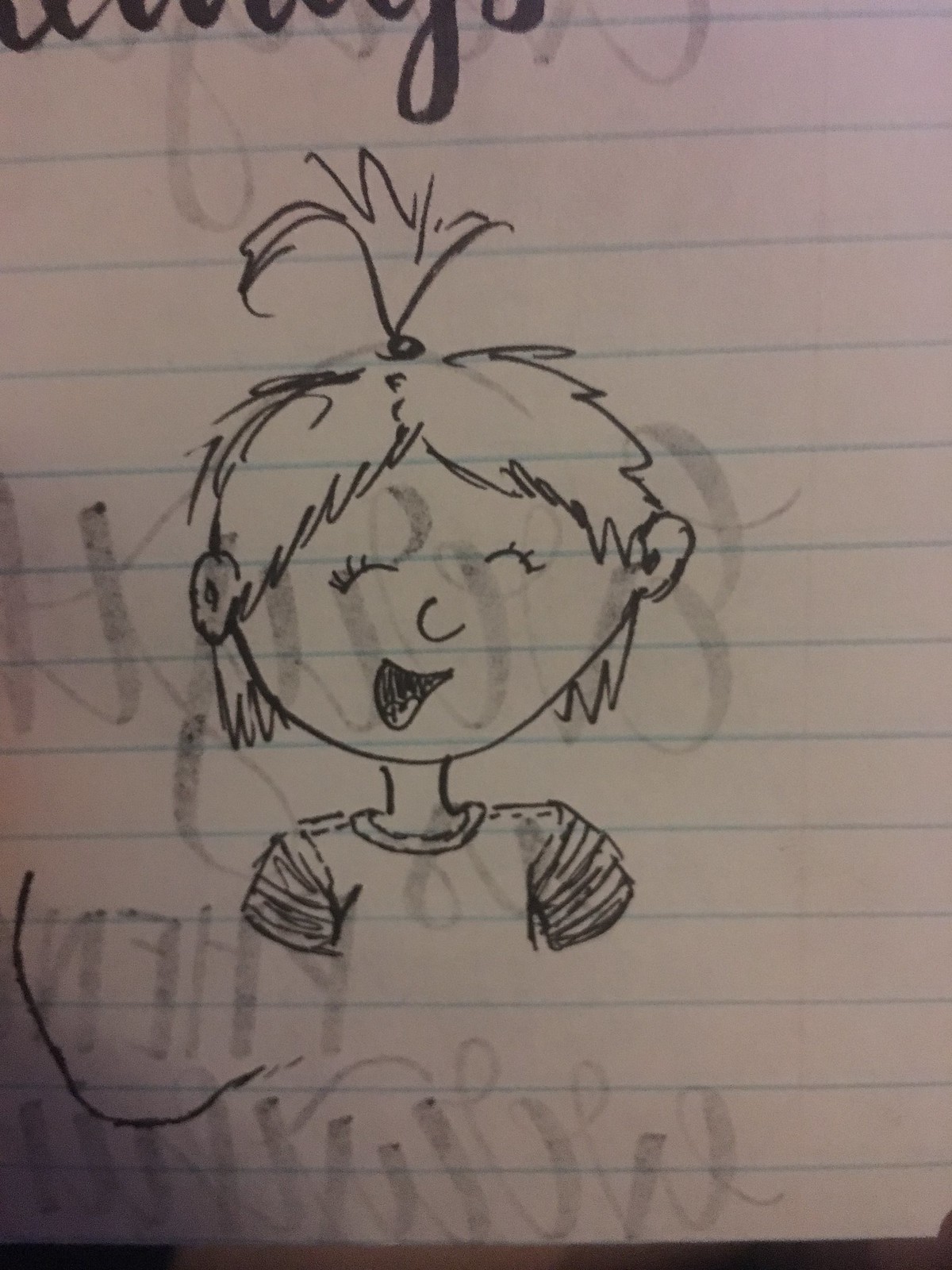The image features a vibrant, cartoonish drawing of a young girl, reminiscent of characters from a Nickelodeon cartoon. She exudes a playful and exuberant demeanor, conveyed through her expressive facial features. Her hair is depicted with a rough, slightly disheveled texture, complemented by a distinctive tuft sticking out at the top, held together by a hairband. The girl's face radiates joy and mischief; her eyes are drawn in an upward slant and appear closed, enhancing her cheeky smile. Adding to her playful expression, she has her tongue sticking out. The visual focus is on the upper part of her body, showcasing her t-shirt and the shoulder area, though her arms are not visible in the image.